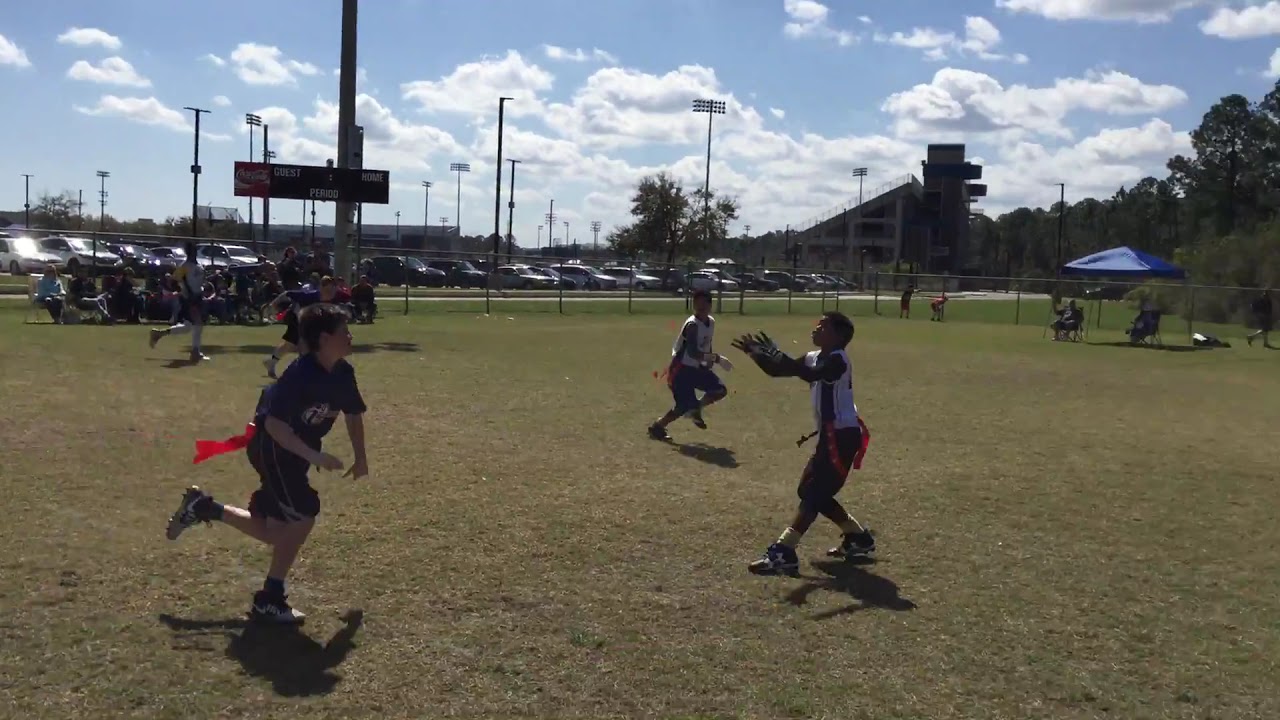The image depicts a lively scene on a grassy field, possibly a baseball or football field, with three children energetically engaged in a flag football game. The grass is a tan color, suggesting fall weather, and the bright blue sky overhead is adorned with white, puffy clouds, creating a stunning backdrop. One child, dressed in a black shirt and black shorts, has their palms open, poised to catch a ball, while the other two children, in white jerseys and black shorts, also appear to be in the midst of a game, each sporting red flags attached to their hips. All the children wear black sneakers. The field is enclosed by a fence, beyond which lies a parking lot filled with cars. Spectators, possibly parents, can be seen on the sidelines, many standing or seated under a blue canopy for shade. Additional features in the background include a scoreboard with 'guest', 'home', and 'period' sections and a Coca-Cola advertisement, along with some buildings and trees to the right, contributing to the overall vibrant and fun atmosphere of the scene.